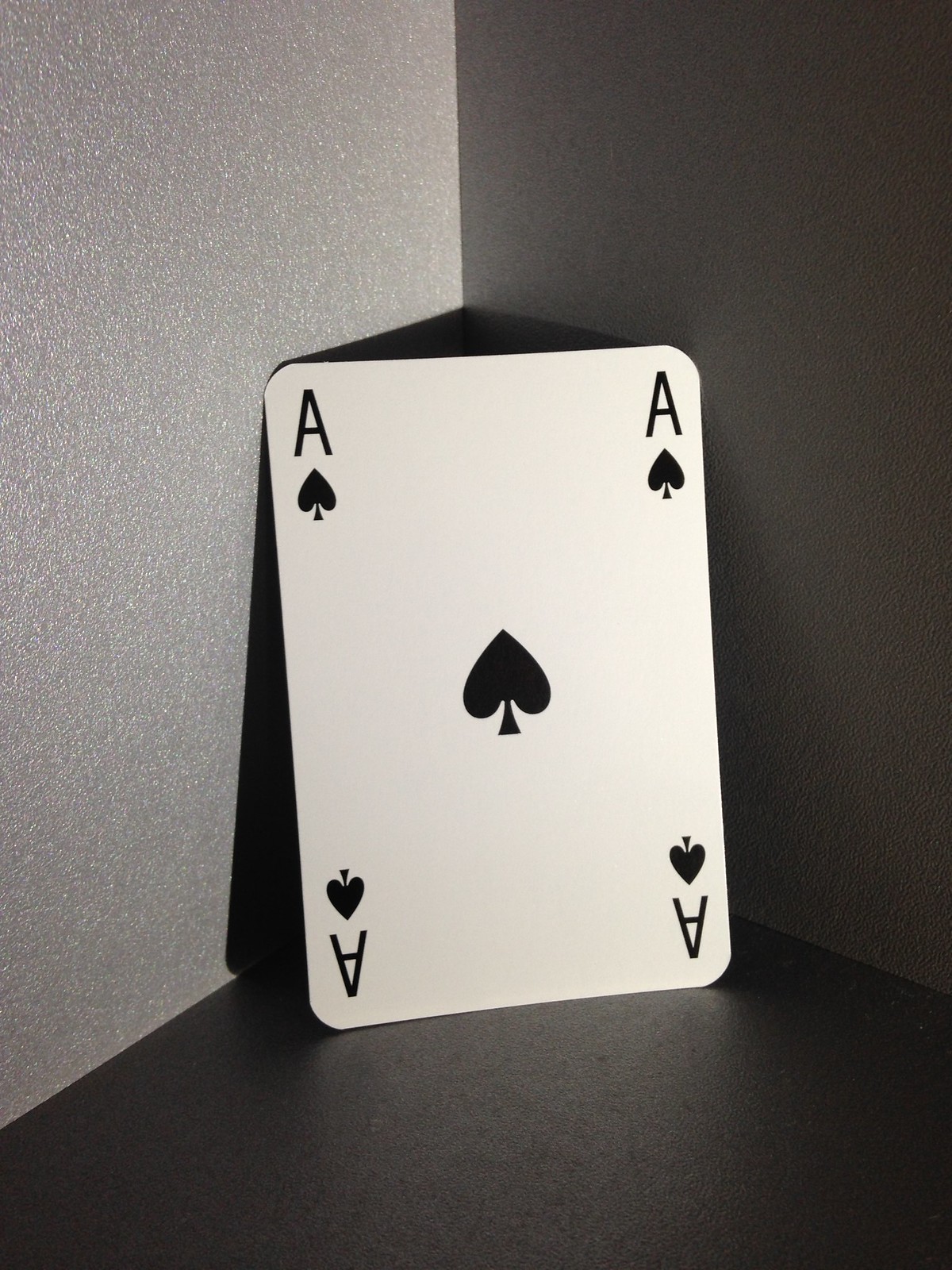The image predominantly features a monochromatic palette, with hues of black, white, and varying shades of grey. Captured at the corner of a wall, the scene presents a black, shiny surface juxtaposed against a wall that transitions from a lighter grey or silver to a darker grey, suggestive of a shadow effect. Centrally positioned against the wall is a playing card—the Ace of Spades—facing the camera. 

The card is a stark white rectangle with gracefully curved corners. Each corner of the card prominently displays an "A," accompanied by a black spade symbol, oriented correctly at the top but inverted at the bottom. Dominating the middle of the card is a larger black spade, perfectly upright. 

The lighting in the image creates a definitive shadow behind the card, implying that the light source is directed either straight at the card or positioned slightly above, casting a distinct, downward-angled shadow.